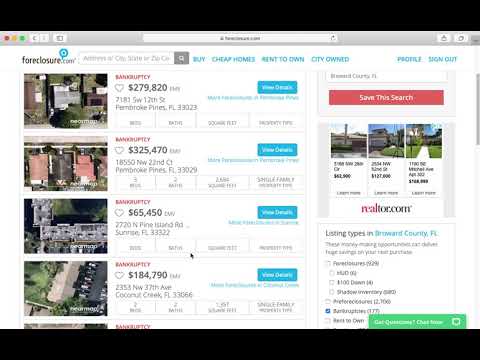The screenshot appears to be taken from a laptop, showcasing an older version of a website viewed in a browser, likely Safari. The webpage displayed is from foreclosure.com, as indicated by the URL and distinctive icons visible at the top, including navigation and sharing options.

The header features a black background with the website name "foreclosure.com" prominently bolded, accompanied by a small house icon in a blue bubble. A navigation bar follows, with options labeled "Buy," "Cheap Homes," "Rent to Own," "City Owned," "Profile," and "Sign Out." Beneath this, a search bar is visible.

To the right of the page, four property listings are displayed, each with details about the foreclosure status, pricing, and location. All properties are marked with "Bankruptcy" in red text:
1. A property in Florida listed at $279,820 with a size of 7,181 square feet.
2. Another in Pembroke Pines priced at $325,470.
3. A home in Sunrise, Florida valued at $65,450.
4. A property in Coconut Creek, Florida at a price of $184,790.

Additional details include a "Save the Search" option in red text, an advertisement for realtor.com, and listing types pertaining to a specific county in Florida, indicated by a clicked option.